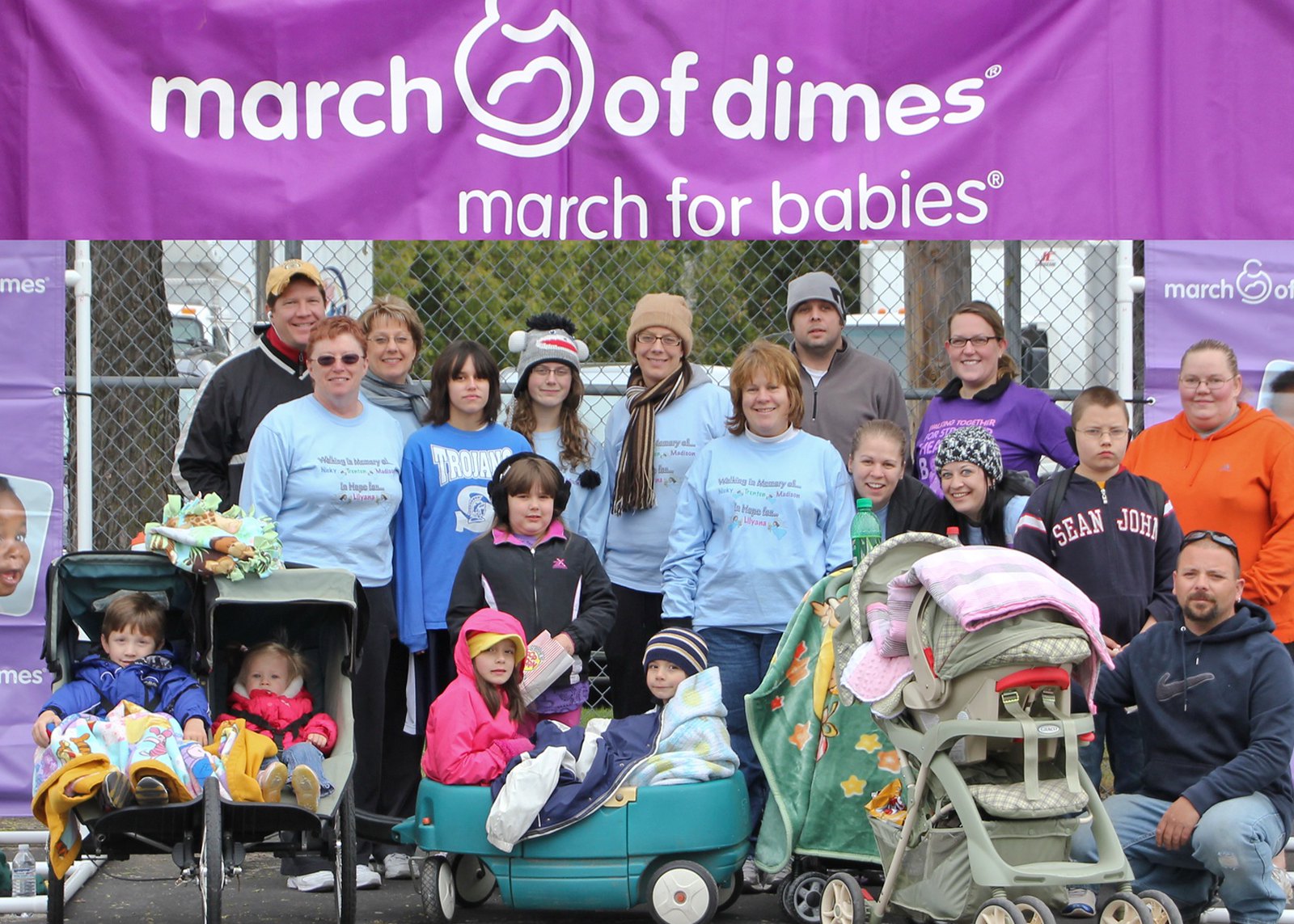In this photo taken at a March of Dimes "March for Babies" walk event, a diverse group of families and friends gather under a prominent purple banner adorned with white text reading "March of Dimes, March for Babies." The banner, showcasing the March of Dimes logo, is affixed above a chain-link fence. The individuals, a mixture of adults, children, and babies, appear to be predominantly white. In the foreground, several strollers and wagons are visible, including a double-wide stroller with two children, a blue wagon carrying two older children, and another stroller partially obscured by a man crouching next to it. Among the group are adults of varying ages, from a 50-year-old man and woman to individuals in their 30s and 40s, who are all dressed in long-sleeve shirts, suggesting a cool climate. The scene captures a moment of camaraderie and joy as the participants pose happily for the photograph.